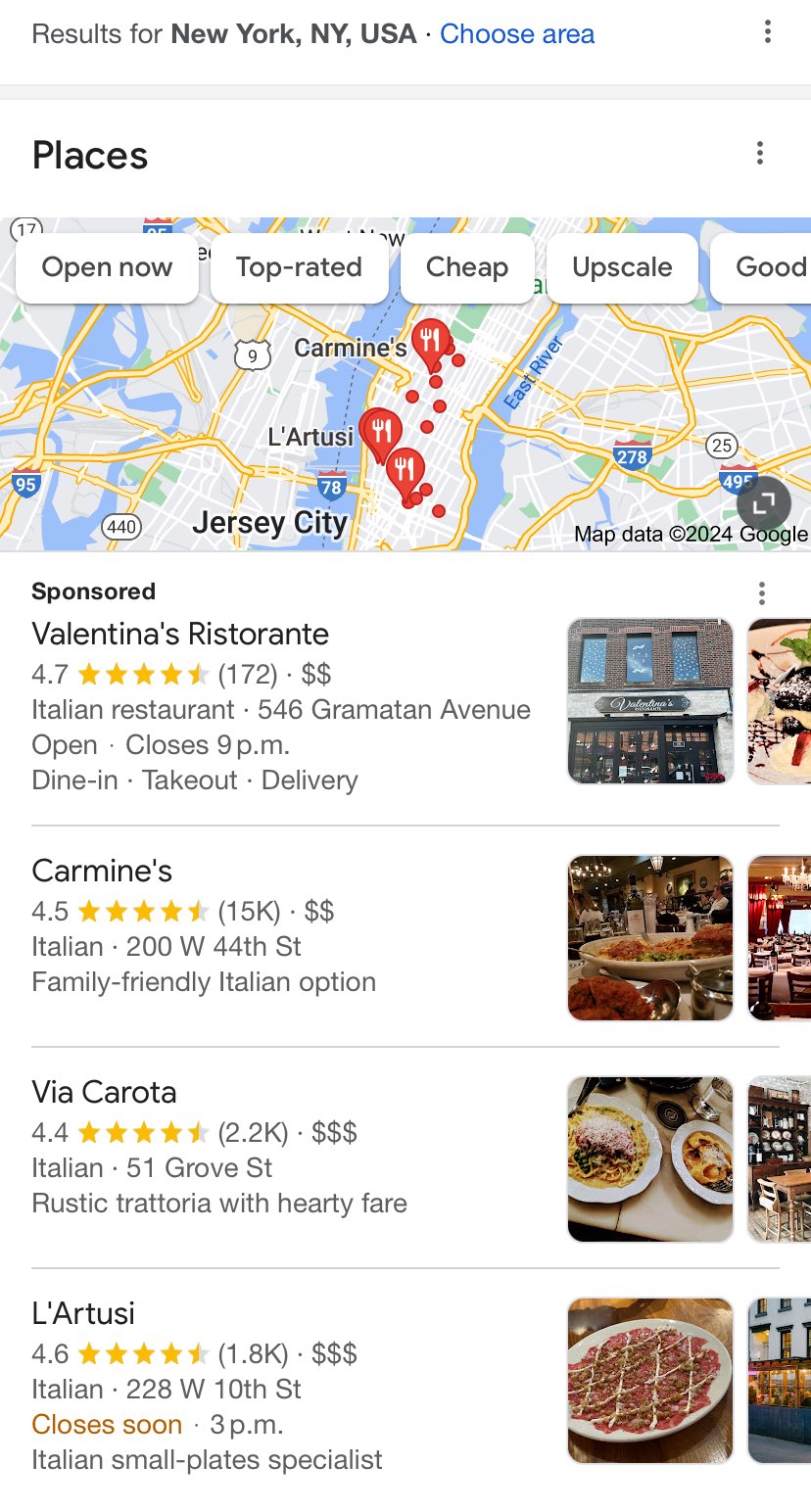On a website showcasing dining options in New York, New York, USA, users are initially greeted with a search result page. At the top of the page, there is an option to "choose area." Below this, there is a section titled "Places," accompanied by a dynamic map with multiple pinpoints representing various restaurants. Each pinpoint on the map can be filtered by different categories such as "open now," "top rated," "cheap," "upscale," and "good."

The first listing on the page is a sponsored restaurant called "Valentina’s Ristorante," an Italian eatery that offers dine-in, take-out, and delivery options. A photograph of the establishment shows a brick building with several windows.

Following Valentina's Ristorante, the next listing is "Carmine's," another Italian restaurant boasting a rating of 4.5 stars. The accompanying image displays a delectable meal served in the dining room.

Next is "Via Carota," with a 4.4-star rating. The visual provided showcases plates of food elegantly arranged on a table, suggesting a charming dining experience.

The fourth listing is "Lartusi," which has achieved a 4.6-star rating. This Italian restaurant, which closes at 3 PM, is represented by an appetizing photograph of a pizza.

This detailed and visually informative layout allows users to conveniently explore and choose from a variety of Italian dining options in New York City.